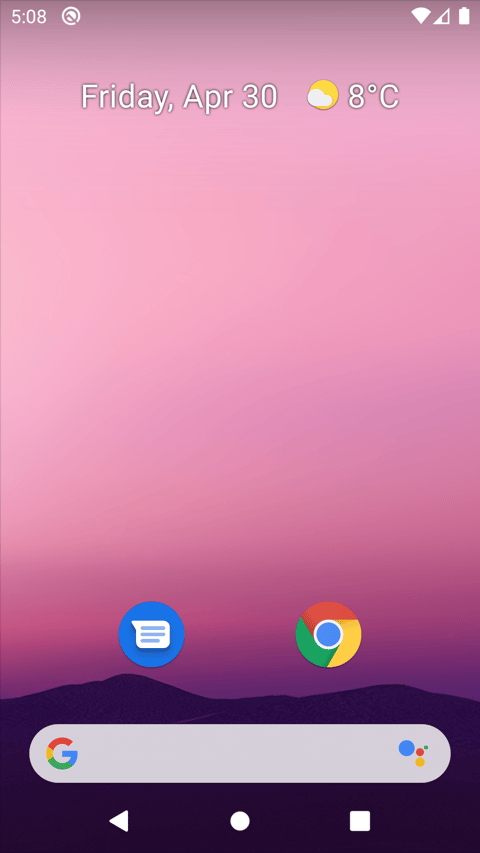This image is a screenshot of a smartphone's home screen. The background image features a stylized, serene landscape with a soft pink sky and mountainous silhouettes, lending a calm and aesthetic appeal. At the top of the screen, notifications display the date and weather: "Friday, April 30th," with a temperature reading of "8°C," indicating a cool day. The time is shown as "5:05," though it is unclear whether it is AM or PM. The battery icon indicates a full charge, suggesting that the phone has recently been unplugged or has not been in use for long.

The home screen is minimalist, featuring only two application icons. The first icon displays the Google logo, commonly associated with Google's suite of services and apps. The second icon is a blue text bubble, which likely represents a messaging or SMS application. Below these icons, there is a Google search bar for quick internet searches, enhancing the screen's functionality without cluttering the space.

Overall, this home screen setup is clean, simple, and efficient, emphasizing essential apps and utilities while maintaining an aesthetically pleasing background.